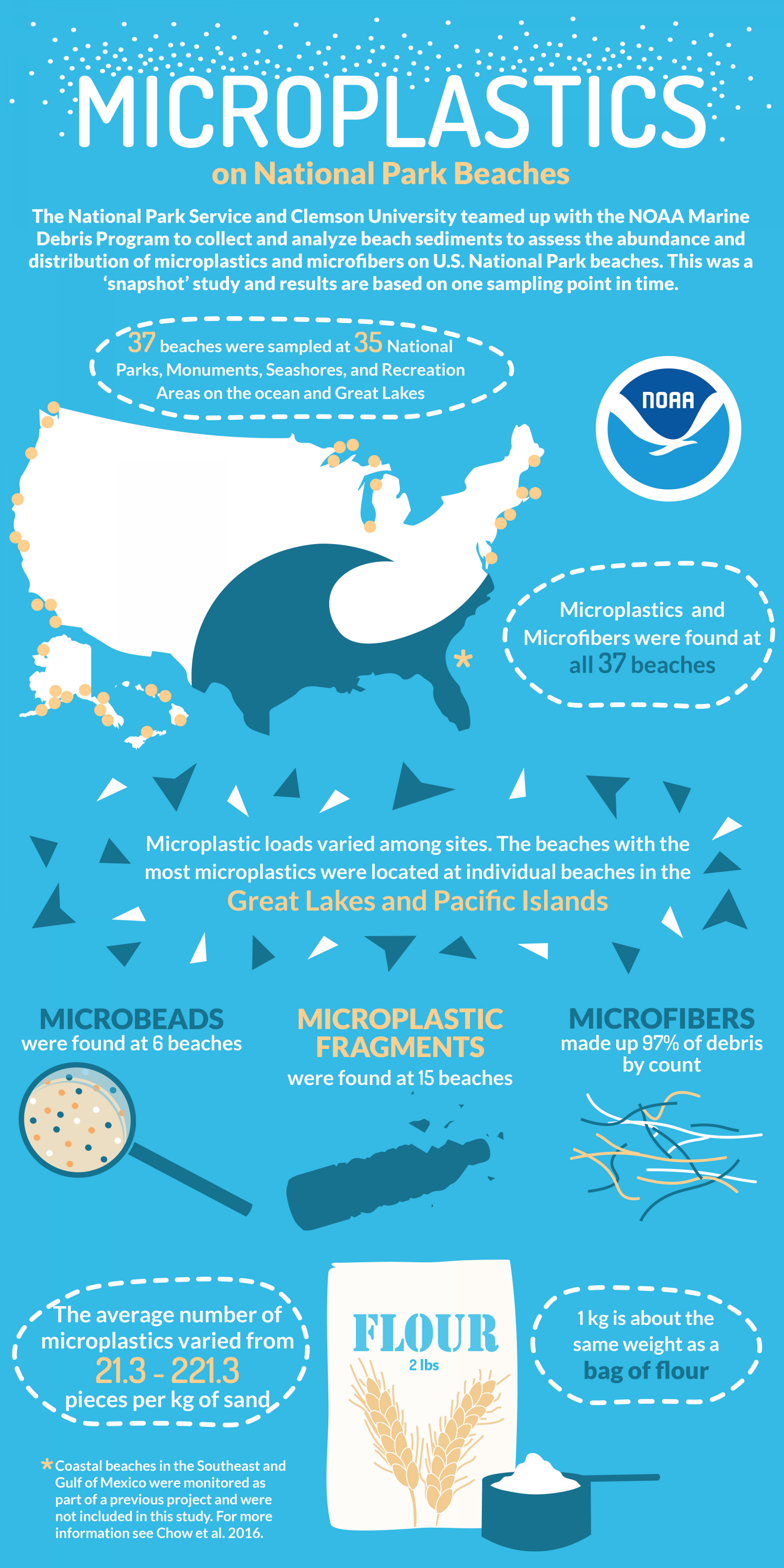The informational graph is a rectangular-shaped poster, three times longer on the left and right sides compared to the top and bottom. It features multiple lines of white and yellow text on a light blue background, accompanied by various graphics to emphasize the text. At the very top, in large white and yellow text, it reads "Microplastics on National Park Beaches." The content below details a collaboration between the National Park Service, Clemson University, and the NOAA Marine Debris Program to collect and analyze beach sediments, assessing the abundance and distribution of microplastics and microfibers on U.S. National Park beaches. This snapshot study's results are based on a single sampling point in time, with 37 beaches sampled at 35 National Parks, Monuments, Seashores, and Recreation Areas across the Ocean and Great Lakes.

The poster highlights that microplastics and microfibers were found on all 37 beaches, with varying loads among the sites. It includes a map of the United States, indicating the locations where the samples were taken, and emphasizes areas with the highest microplastic concentrations like the Great Lakes and Pacific Islands. Below the map are diagrams illustrating different types of microplastics: a magnifying glass labeled "microbeads," bottles labeled "microplastic fragments," and fibers labeled "microfibers." Additionally, a drawing of a box of flour is included, possibly for scale or comparison.